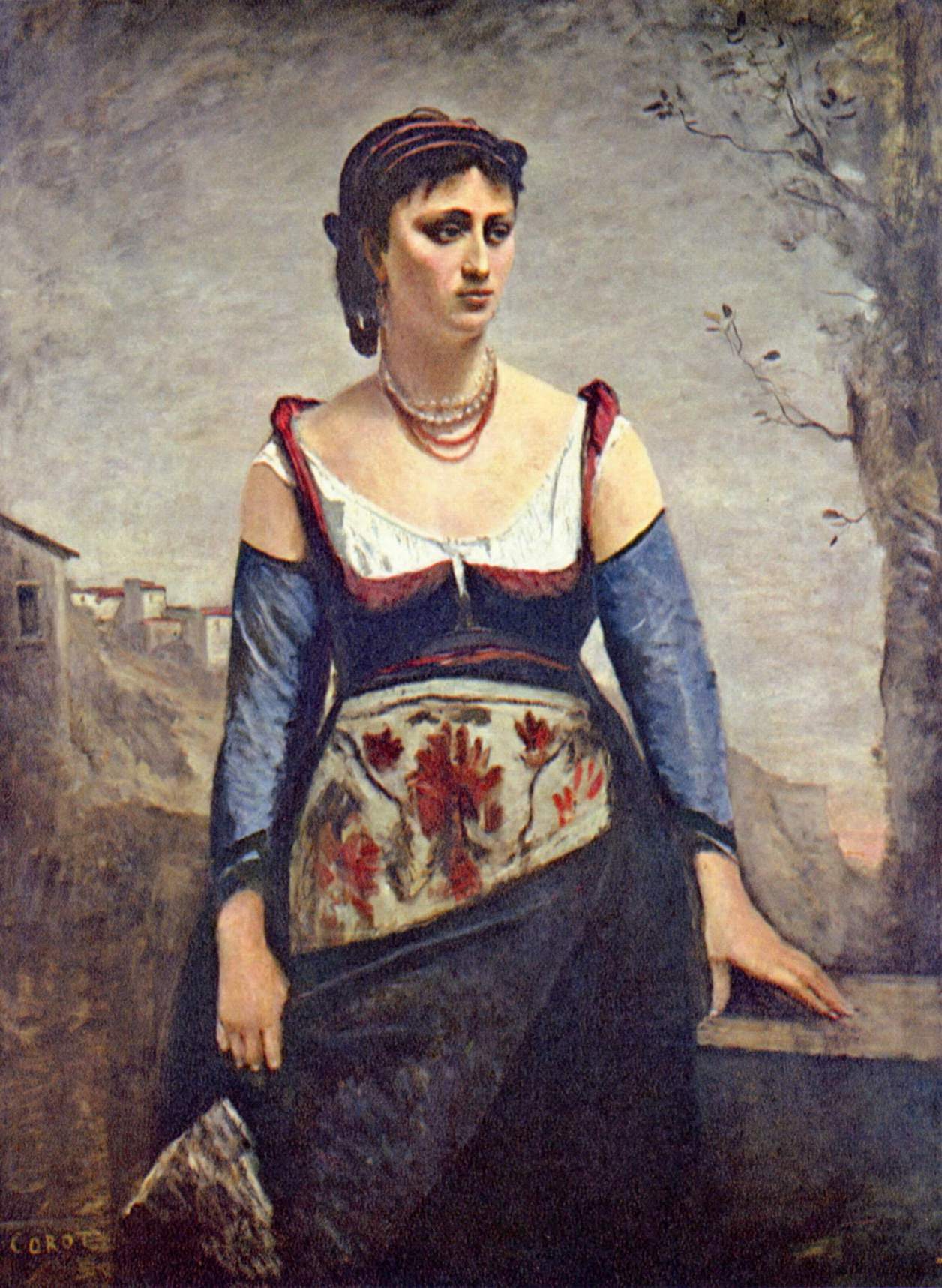The painting depicts a young, somber-looking woman standing in the forefront, her body visible up to her knees. She is adorned in a detailed dark blue dress with a wide, long skirt, a white undershirt, and striking red shoulder straps. The front of her dress features a cream-colored apron beautifully embellished with red floral patterns, which she is holding delicately. Her neck is adorned with a double-strand pearl necklace and a double-strand red necklace. Her black hair is neatly braided and interwoven with various red ribbons. Behind her lies a small, picturesque town composed of white buildings with red roofs, nestled against what appears to be a mountainside or hillside. To the right of the woman stands a weathered brown tree trunk. The sky dominates much of the background, painted in a light gray with hints of red near the bottom right, adding a touch of dusk or dawn to the scene. The woman gazes slightly to the right, her face reflecting a subtle sadness.